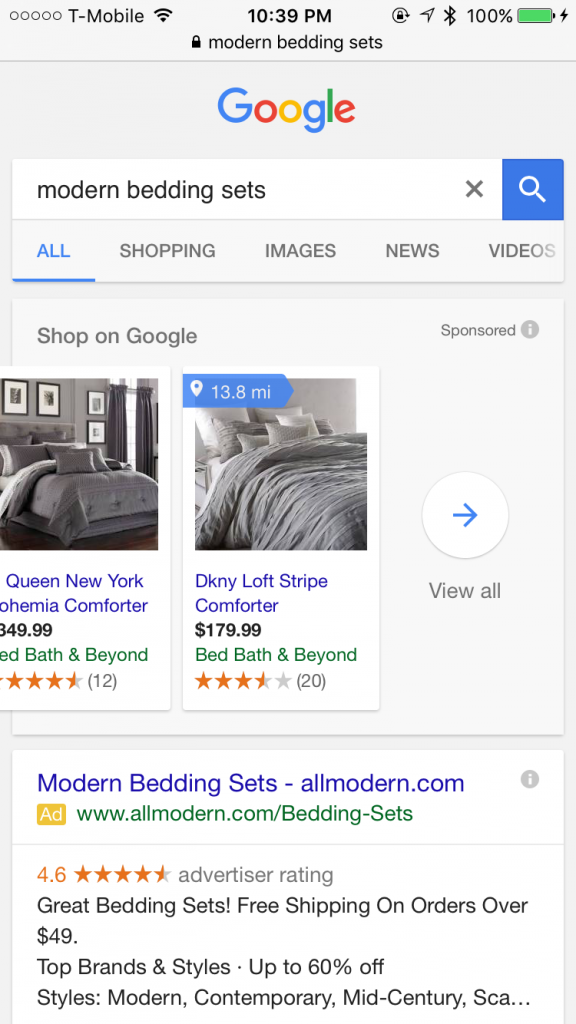The image is a vertical screenshot taken on a cell phone, displaying an online shopping search result for "modern bedding sets." 

- **Top of the Screen:**
  - **Upper Left Corner:** The status bar shows T-Mobile network with active Wi-Fi in black icons.
  - **Center:** The time is displayed as 10:39 p.m. in black text.
  - **Upper Right Corner:** The Bluetooth icon is lit, and the battery is fully charged at 100%.

- **Search Interface:**
  - Just below the status bar, small black text reads "modern bedding sets."
  - A light gray banner features the word "Google" centered, with a search bar underneath showing the query "modern bedding sets."

- **Search Results:**
  - At the top, "Shop on Google" is written, with the term "Sponsored" in small gray text to the right.
  
  - **First Search Result (Left Image):**
    - Shows a bedroom with a gray bedding set.
    - The product name is displayed in blue text: "Queen New York Comforter."
    - "Bed Bath & Beyond" is written in green text, accompanied by "12 reviews."

  - **Second Search Result (Right Image):**
    - Shows another bedroom with gray bedding.
    - The product name, "DKNY Loft Stripe Comforter," is in blue text.
    - Below it, the price is listed as "$179.99" in black text.
    - "Bed Bath & Beyond" is again displayed in green text.

Overall, the screenshot captures the details of a Google Shopping search page, highlighting modern bedding set options from Bed Bath & Beyond.